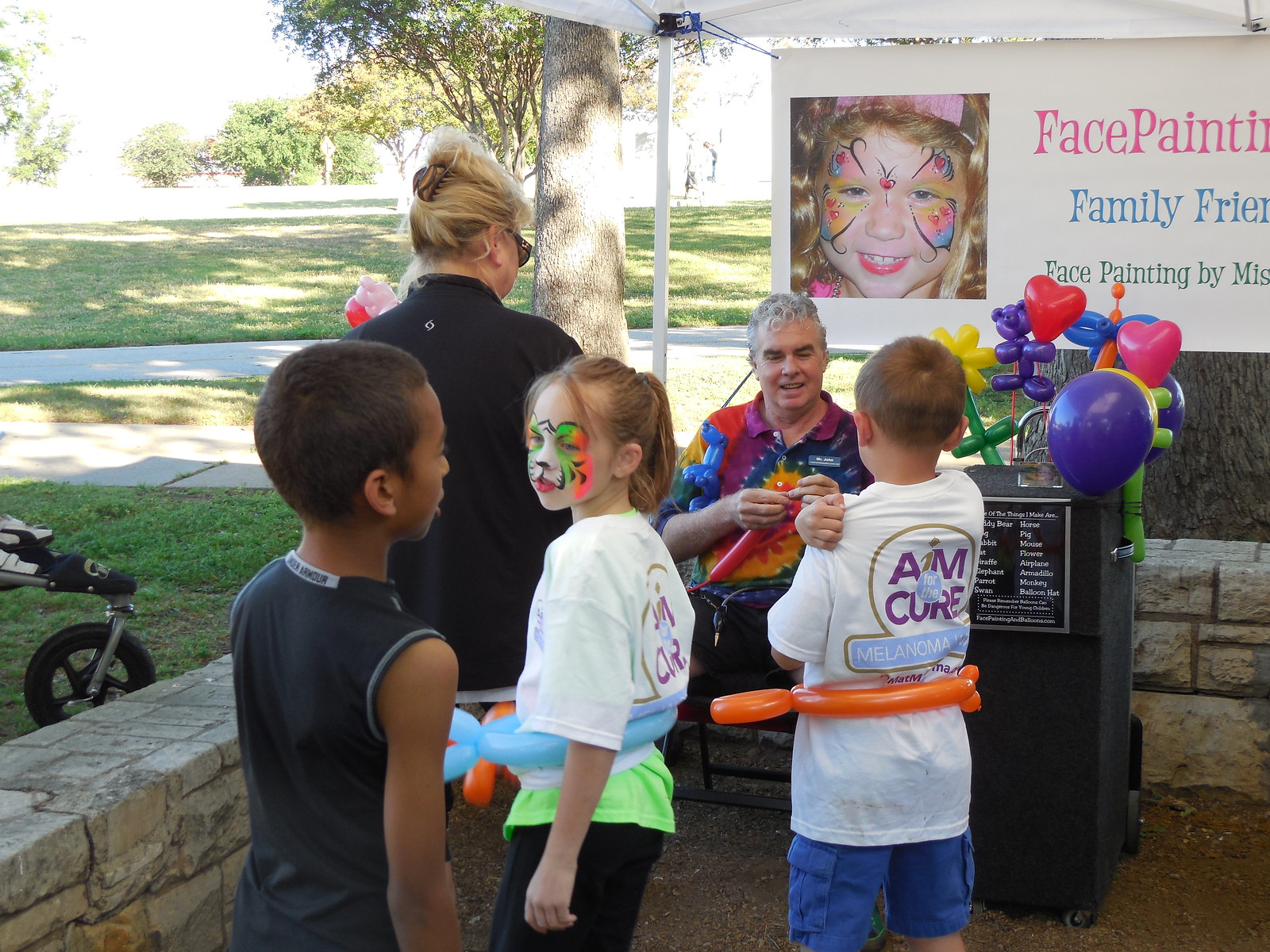This image, taken on a bright day in what appears to be an early spring or summer festival at a park, captures a lively scene of children eagerly waiting to have their faces painted. The foreground features three children; two boys and a girl. One boy on the left, possibly of Indian descent, is dressed in a sleeveless black t-shirt and dark shorts. The other two children, of European descent, have blonde hair and are wearing white t-shirts that say "Aim a Cure" and "Melanoma," suggesting the event is a charity function. One of these boys, sporting a white t-shirt and shorts, stands on the right. Between them, a young girl with tiger face paint looks curiously at the boy behind her. 

To the right of the children stands a woman with blonde hair tied in a bun, wearing glasses and a black top, engaged in conversation with an older man sitting in front of a helium tank, creating balloon animals. This man, who has gray hair and is dressed in a colorful tie-dye shirt, is tying balloons into shapes for the children. Surrounding him is a vibrant assortment of balloons in colors of blue, red, yellow, and green, crafted into various forms like animals, flowers, and hearts. 

Behind him is a white banner marred by a partial view, reading "Face Painting" in pink letters with a picture of a girl who has had her face painted. Below this, there are additional words in blue and green fonts, partially readable as "Family Friend" and "Face Painting by Ms." The picturesque background reveals a low stone wall, a lush green lawn, and an array of trees, further emphasizing the outdoor, festive atmosphere.